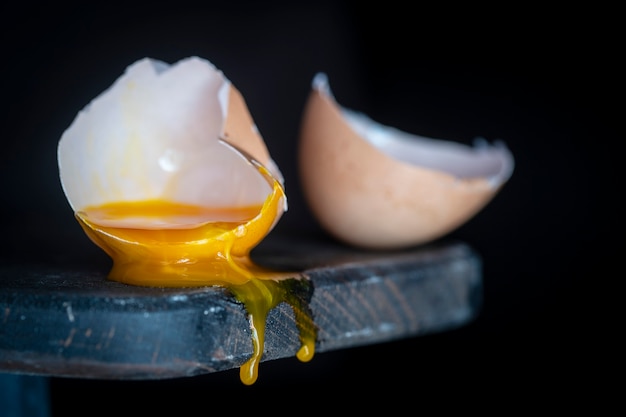The image showcases a visually compelling scene: against a black background, there is an aged, possibly wooden stand that appears bluish-green due to wear, adorned with whitish-brown markings. This stand serves as the base for two cracked eggshell halves. The outer surfaces of these shells are light brown or tan, while their interiors are white. One eggshell in the foreground contains a vivid yellow yolk that has broken open, causing the yolk to spill out and cascade down the stand, forming droplets that seem to edge towards the floor. The other eggshell half is situated slightly behind and to the side, appearing empty in contrast. The focused lighting and composition emphasize the textures and colors, making the aged, bluish stand and the contrasting egg elements stand out vividly.